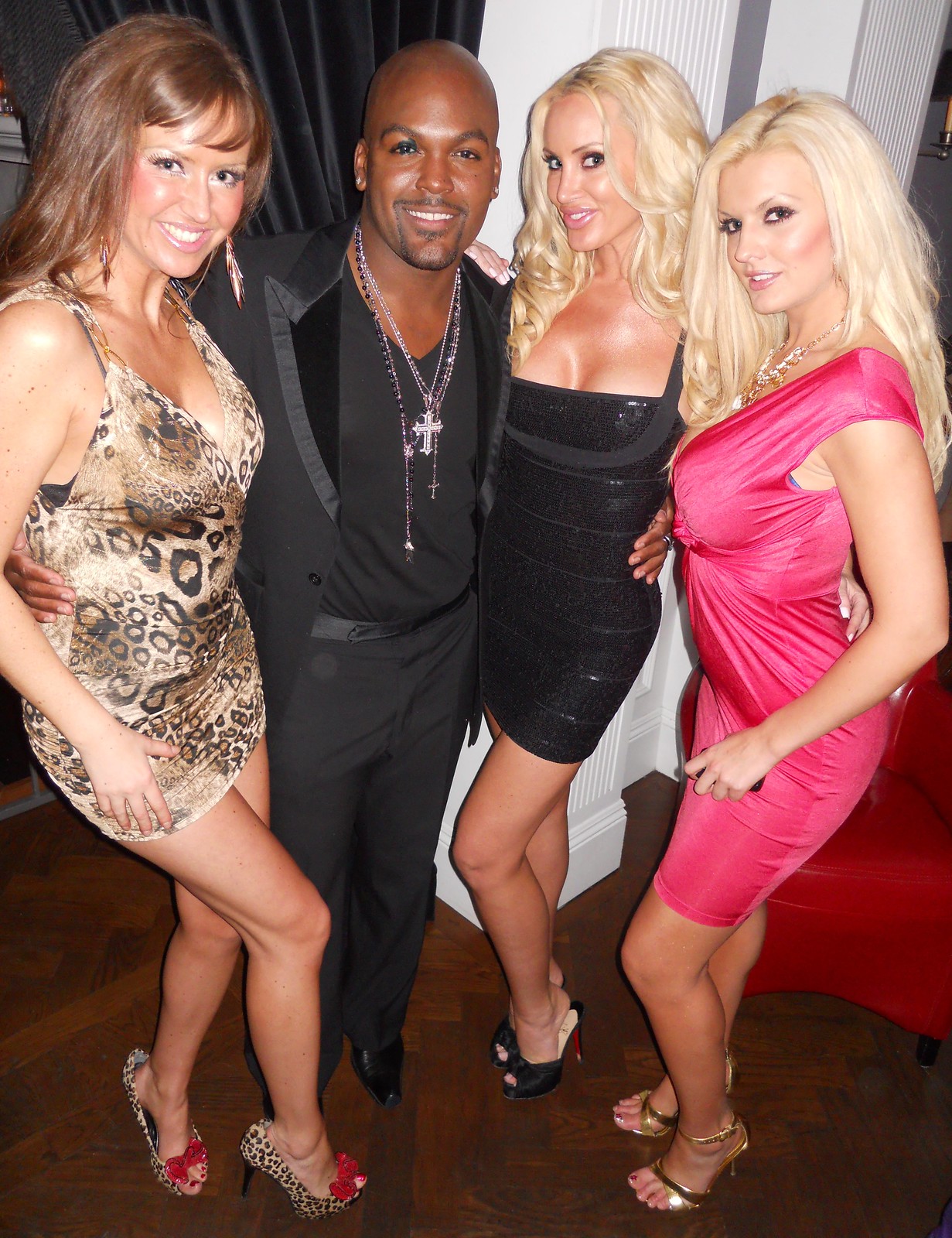In the image, a stylishly dressed black man stands in the middle, surrounded by three elegant white women. The man, sporting a black suit with satin detailing and velvet lapels over a black shirt and pants, accessorizes with multiple silver necklaces, including one with a cross, a goatee, and subtle eye makeup on one eye. His arms are wrapped around the women flanking him on either side.

To his left, a woman with brown hair and bangs wears a tight, short, brown and black cheetah print mini dress paired with matching high heels adorned with red bows. She has heavy makeup on and a confident smile. 

To his right, two blonde women strike a pose. The nearer woman dons a black, form-fitting mini dress that accentuates her cleavage, and completes her look with black stilettos. The farthest woman from the man is dressed in a hot pink satin mini dress, looking slightly ill-fitting, and is accessorized with a necklace and gold high heels.

All four are posing with smiles and slightly bent knees in an attractive stance, standing on a dark brown hardwood floor. The background includes a red chair, white pillars, and black curtains, setting an elegant yet lively atmosphere fitting for a party or special event.